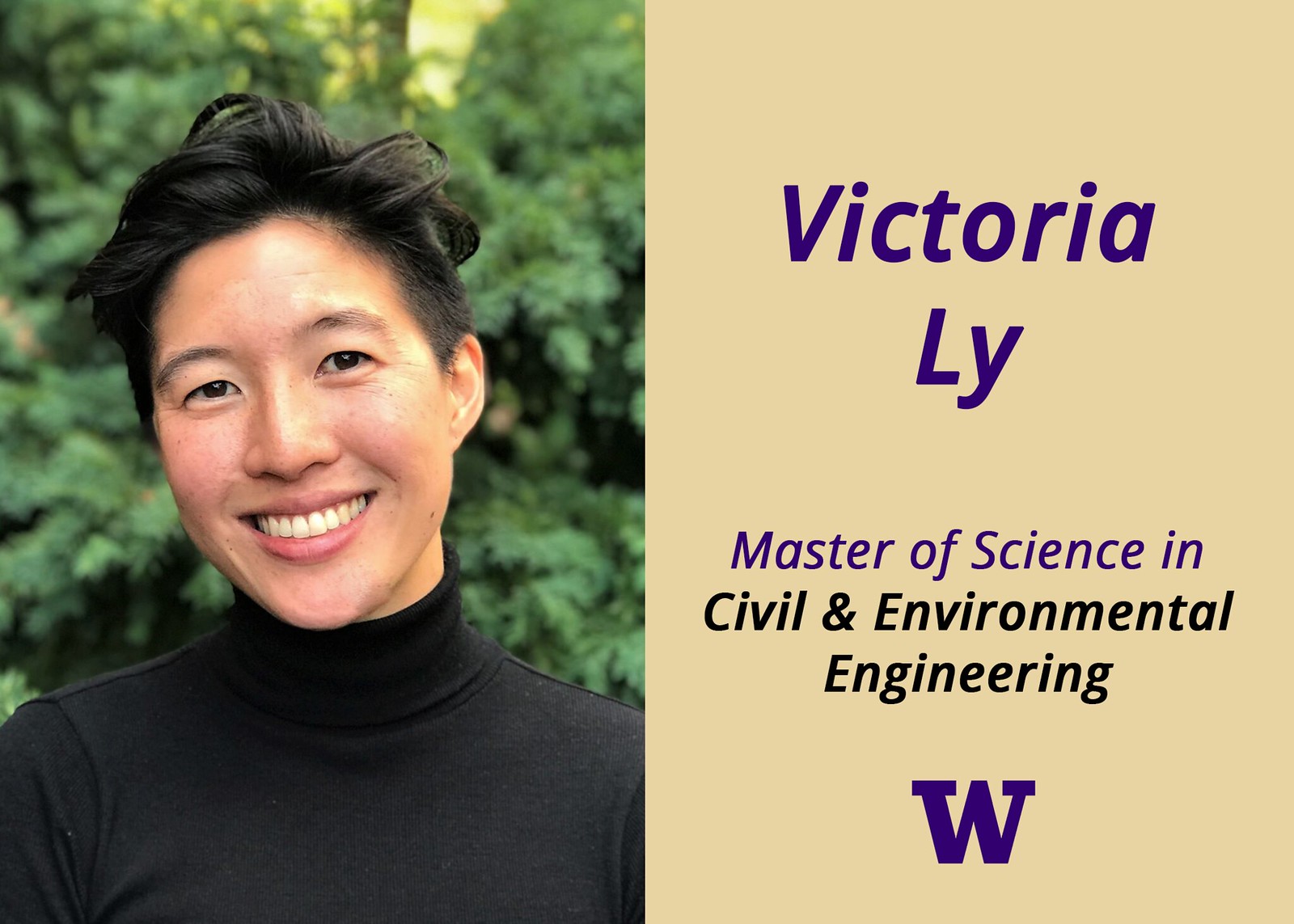The image is a professionally designed split-screen presentation of Victoria Lee, showcasing her academic achievements. The left side features a close-up portrait of Victoria Lee, an Asian woman with black hair that is styled shorter on the sides and top. She is smiling warmly at the camera, wearing a black top with a higher neckline. The background behind her is blurred vegetation, suggesting she is outdoors. The right side of the image has a tan background with purple text that reads "Victoria Lee, L-Y." Below that, it states "Master of Science in Civil and Environmental Engineering." A bolded blue 'W' symbol is also present, representing the University of Washington.